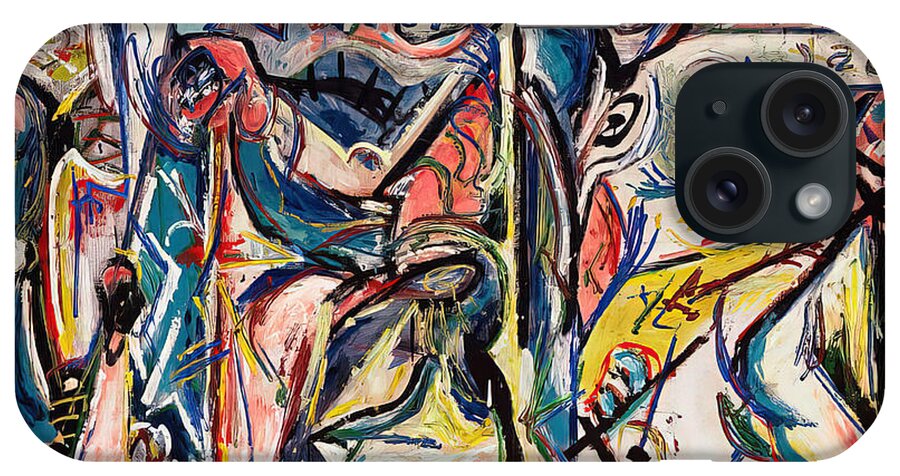This photograph displays the back of an iPhone encased in a colorful, abstract art-style case. The case features a myriad of colors including yellows, blues, pinks, greens, whites, reds, and golds, creating a chaotic yet hand-painted appearance with black lines running throughout the design. The phone's camera area, positioned in the top right corner, is a black square with two camera lenses and a small microphone. The vivid case contrasts sharply against the pristine white background, making the artful design stand out even more. There are no other objects in the image, focusing attention solely on the iPhone and its unique case.